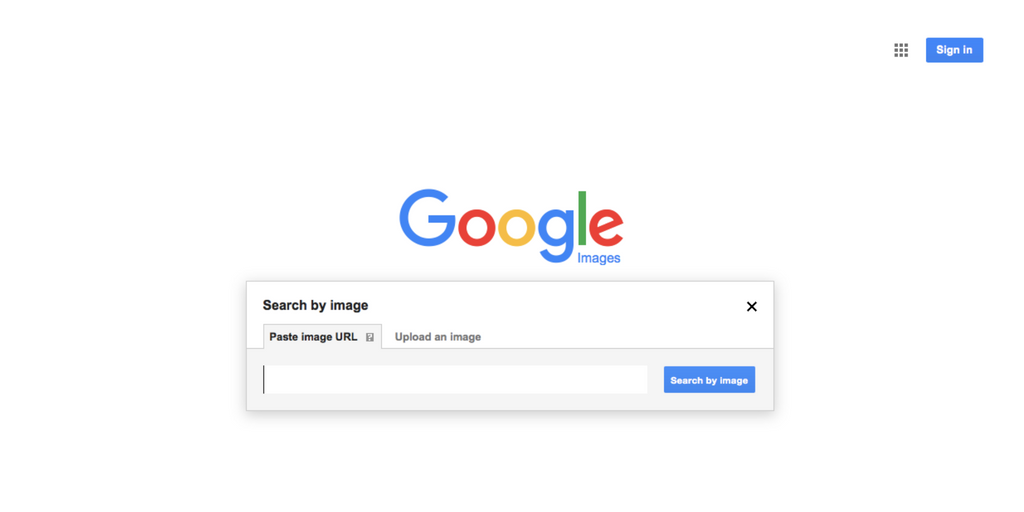The screenshot features a predominantly white background with various elements positioned throughout the page. In the top-right corner, there is a charcoal gray or black square icon made up of nine smaller squares arranged in a 3x3 grid. Adjacent to this icon is a blue tab that reads "Sign in" in white text, with both the "S" capitalized.

Centrally displayed is the iconic "Google" logo, characterized by a capitalized 'G' in blue, followed by the first 'o' in red, the second 'o' in yellow, the 'g' in blue, the 'l' in green, and the 'e' in red. Beneath the Google logo, the word "Images" appears in blue text with a capital 'I.'

Midway down the page, a pop-up banner reads "Search by image" on a white background. To the right of this banner, there is an 'X' icon for closing the pop-up. "Search" is written with a capitalized 'S.' Further down, in light gray text, the banner prompts the user to "Paste image URL," with 'URL' fully capitalized. Below this prompt, there is an input bar where the URL can be pasted, accompanied by a blue tab that also says "Search by image" in white text.